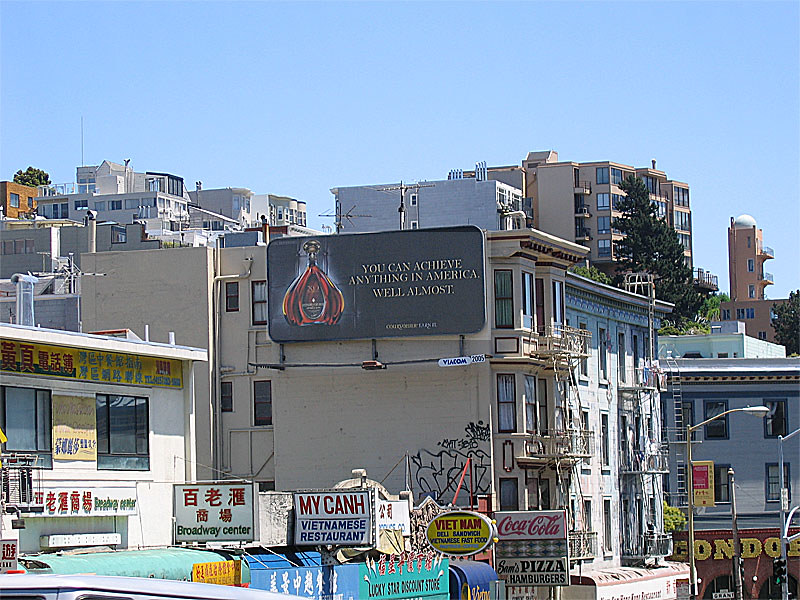Captured in broad daylight, this cityscape features an eclectic mix of urban architecture. At its heart, a rectangular billboard commands attention. Mounted on the side of an apartment building adorned with graffiti, the billboard is black with bold, lighter-colored lettering that reads, "You can achieve anything in America... well, almost." An illustrated bottle accompanies the lettering, adding an intriguing visual element. 

The apartment building presents a stark front with multiple windows and traditional fire escape ladders. Surrounding it, an assortment of buildings of varying heights stretch into the distance, most built from brick and punctuated by numerous windows. Closer to the viewer, a vivid array of signs adds vibrancy to the scene, including notable mentions like a Coca-Cola sign, adverts for "Pizza & Hamburgers," "Vietnam Deli," and "My Can Vietnamese Restaurant." prominently displayed above the bustling "Broadway Center." The combination of these elements paints a dynamic picture of urban life and the rich tapestry of a bustling cityscape.